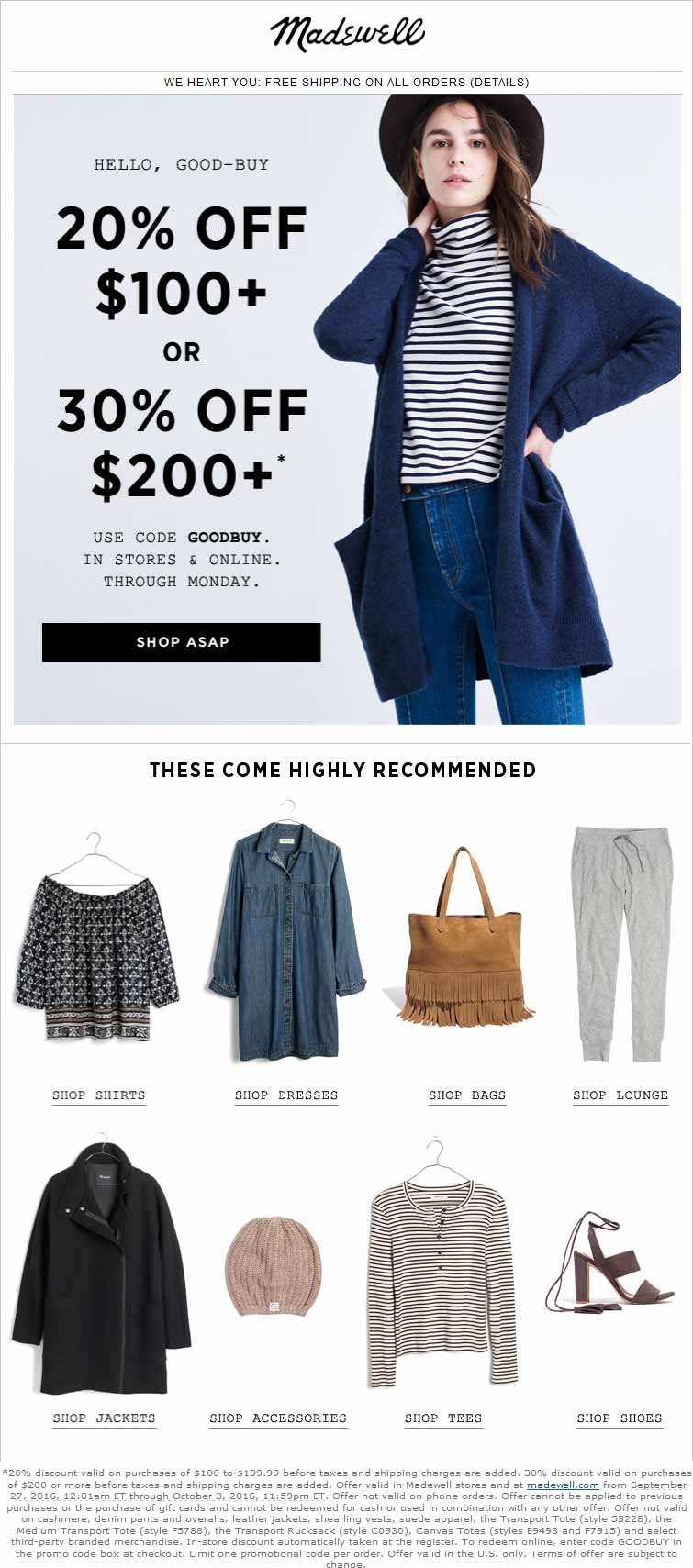This image shows the interface of the Madewell app or website with a predominantly white background. At the very top, the word "Madewell" is displayed in a cursive font. Below it, in very small letters, it reads "We heart you: Free shipping on all orders (details)".

Positioned beneath this text is a small box with a light purple background, featuring an advertisement banner with a woman posing. To the left of her, the banner promotes a discount: "Hello Goodbye: 20% off $100 and more, or 30% off $200 and more. Use code GOODBUY in stores and online through Monday." Below this promotion is a small black button labeled "Shop ASAP".

Underneath the banner, a white section features text that says, "These come highly recommended", accompanied by images of various products. Each image is paired with a corresponding call-to-action button. From left to right, the sections are: "Shop Shirts" (shirts), "Shop Dresses" (dresses), "Shop Bags" (bag), "Shop Loungewear" (loungewear), "Shop Jackets & Accessories" (jackets and accessories), "Shop Tees" (tees), and "Shop Shoes" (shoes).

At the very bottom, fine print provides additional details about the discounts and purchasing requirements.